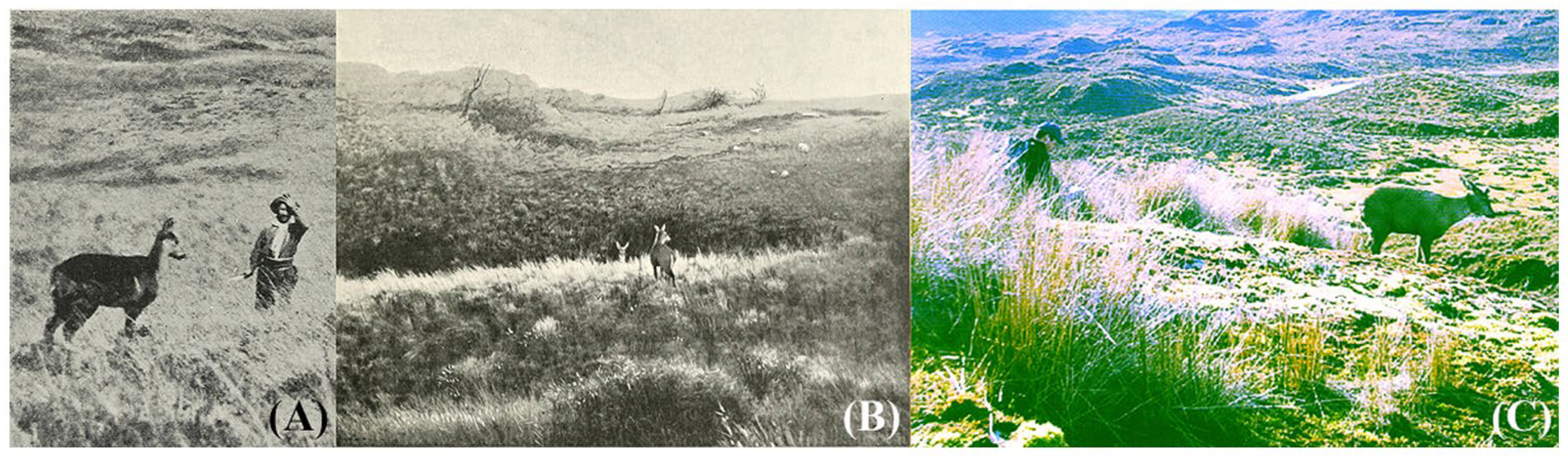The image consists of three photographs placed side-by-side, each labeled with a letter in parentheses at the bottom right corner: A, B, and C. The first photograph (A) on the left is the smallest and done in black and white. It depicts a man standing in a grassy field on the right side, with one hand over his head, and a scraggly-looking deer on his left. This photograph has a vintage look with the man dressed in old-fashioned attire. The middle photograph (B), also in black and white, shows a field with a couple of hills and two deer. The largest photograph (C) on the right features a color-distorted scene of green, yellow, white, and blue hues. It presents a hillside with a man possibly holding a camera on the left and a deer or elk with a collar around its neck standing to his right. The images offer a varied look at humans and deer in different settings.